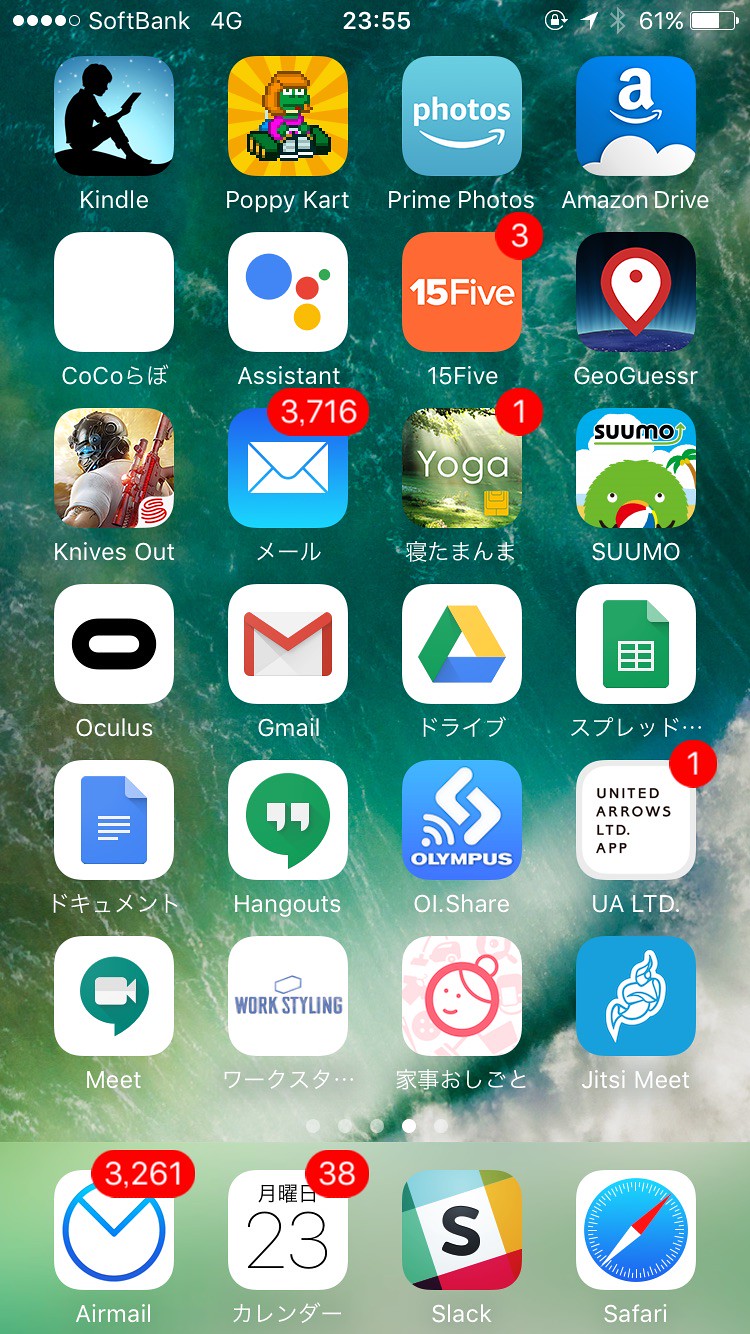The image is a screenshot of a smartphone's home menu page displayed in military time, showing "23:55" at the top with white font. The status bar indicates that the phone battery is at 61%, Bluetooth is enabled, location services are active, and rotation lock is on. In the top left corner, four out of five white signal dots are visible alongside "Softbank" and "4G."

The background features serene ocean waves. The app icons are organized in a grid, starting from the top left with Kindle. Next in line are Poppy Cart, Prime Photos, Amazon Drive, Coco, and an app with Chinese characters. Additional apps in the sequence include Assistant, 15-5, GeoGuess, Knives Out, Mail, Yoga, Sumo, Oculus, and Gmail. 

Following these, there are more apps with Chinese characters, an app that resembles Google Photos, a green icon app, and Notebook. 

At the bottom of the screen, the dock holds four primary apps: Safari, Slack, Calendar, and Air Mail.